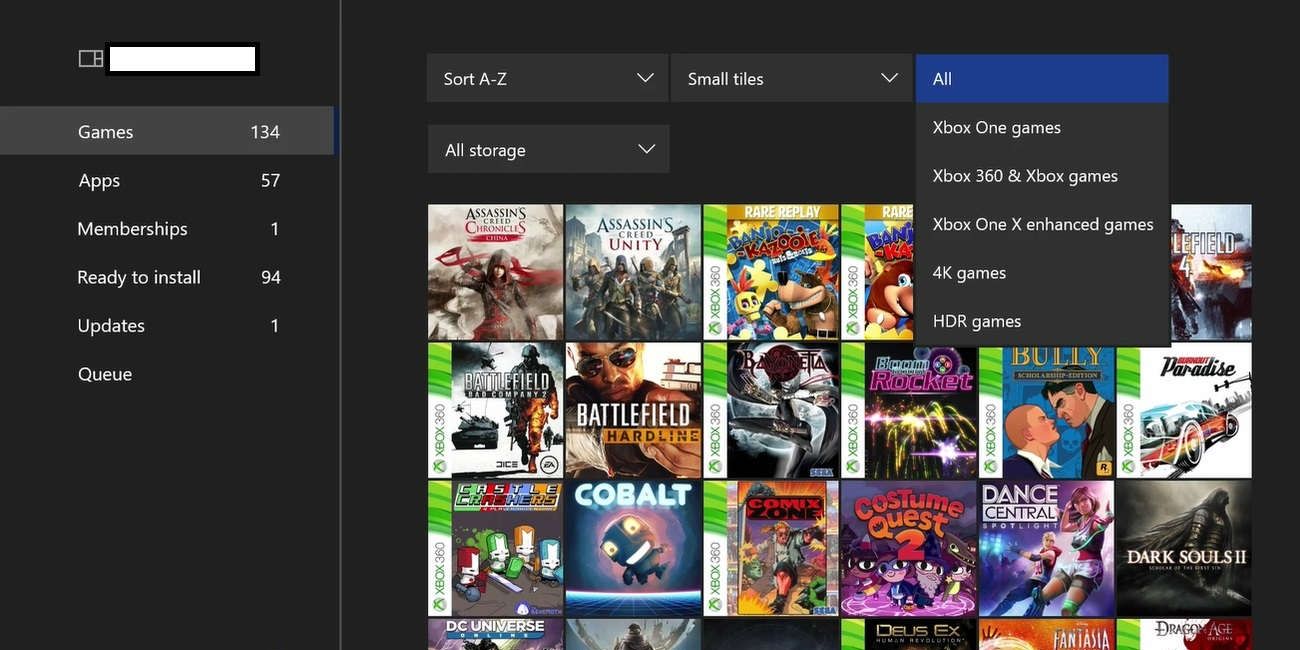The image appears to be a screen capture from an Xbox gaming interface, likely showcasing the user's game library or an online gaming site. The background is predominantly black, providing a sleek and modern look to the interface. On the left side, there is a sidebar with a white box icon resembling a television set, accompanied by several submenu items. These submenus include: "Games" (134), "Apps" (57), "Memberships" (1), "Ready to Install" (94), "Updates" (1), and "Queue."

In the middle portion of the image, there are sorting options, including "Sort A to Z" with a dropdown menu and an option for "Small Tiles" also with a dropdown arrow. The category "All" is highlighted in a blue box with white text. The subsequent labeled categories in white text are: "Xbox One Games," "Xbox 360," "Xbox Games," "Xbox One X Enhanced Games," "4K Games," and "HDR Games." Additionally, there is a box labeled "All Storage."

The image also features a diverse array of game graphics arranged in a mosaic layout. Some of the highlighted games include:

1. **Assassin's Creed** - Depicting a battle scene with a red and gray figure.
2. **Assassin's Creed Unity** - Showcasing warriors dressed in gray and olive, with a red and blue title.
3. A variety of animated characters including:
   - A cartoon dog.
   - A cartoon bird.
   - A cartoon monkey.
4. **Battlefield Games** - Two graphics, one featuring a soldier and another showing a person in sunglasses holding a gun.
5. A game with gray and red hues.
6. A game in blue, pink, and black tones.
7. **Bully** - Illustrating two men staring at each other angrily.
8. **Paradise** - Featuring a car.
9. **Castle Something** - Displaying red, green, gold, and blue cartoon characters.
10. **Colbot** - Showing a small black robot with yellow eyes and a big smile.
11. **Comic Zone** - Featuring a blonde-haired figure.
12. **Costume Quest 2** - Highlighting superheroes and a little wizard cartoon character.
13. **Dance Central**
14. **Dark Souls 2** - Depicting a robed figure in black.
15. Several other games at the bottom of the image, where the colors are distinguishable but the full names are not clearly visible.

This detailed interface design reflects an organized and visually engaging way for users to navigate and explore their game library.